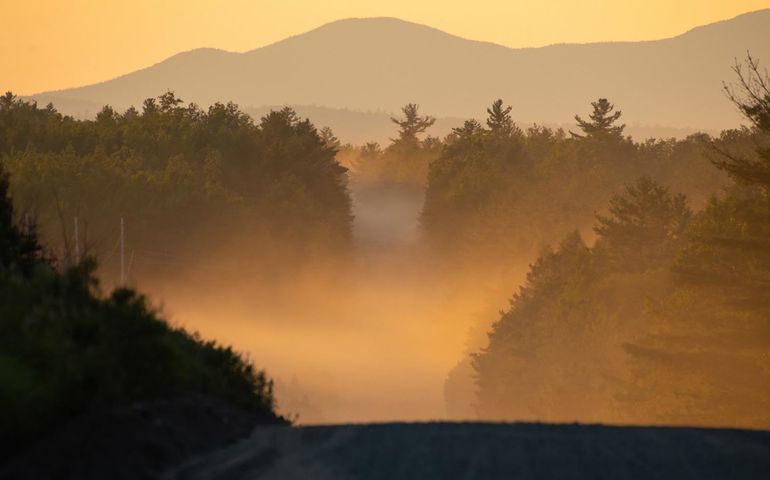The photograph, rectangular in shape and approximately 5 to 6 inches wide by 4 inches high, captures a serene scene at sunset. Dominating the lower part of the image, a dark, flat road appears to stretch out before dipping down a steep hill, creating an illusion that it ends abruptly. This descent into the valley below is enveloped in dense, orange-yellow fog, likely colored by the soft light of the setting sun. On either side of the road, the landscape is densely packed with trees, their tops barely visible through the thick mist that rises from the unseen depths. A small green brush-covered hillside can be seen on the left, adding to the sense of depth in the image. In the far background, a hazy, gray mountain range stands under an orangish-yellow sky, completing this ethereal landscape.